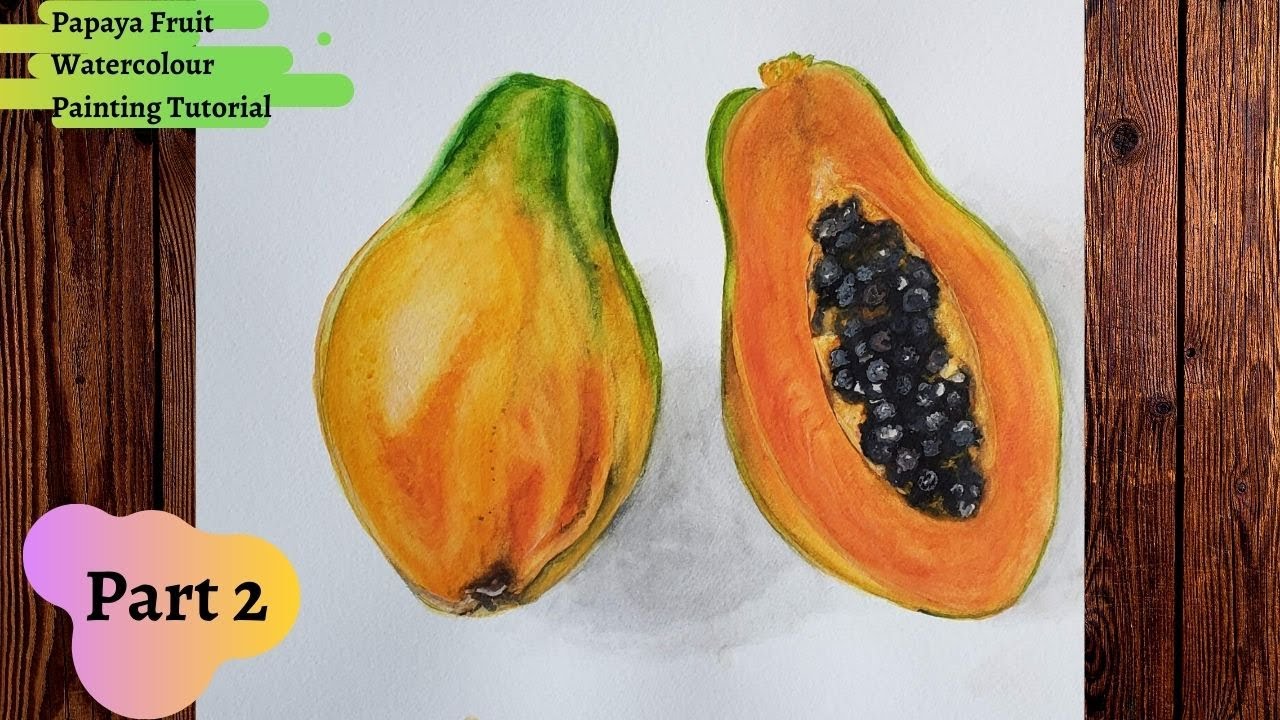This image depicts a detailed watercolor tutorial on painting a papaya, positioned on a sheet of white watercolor paper which covers most of the medium to dark, walnut-colored wooden background. The watercolor paper occupies approximately two-thirds to three-quarters of the image from top to bottom and features a header on the top left corner that reads, "Papaya Fruit Watercolor Painting Tutorial," with "Part 2" indicated below.

The painting showcases a whole papaya on the left side of the paper, illustrating its light green and orange skin with a brown-black tip where the stem was attached, and a sliced half on the right, revealing the vibrant orange flesh and clustered black seeds with white highlights at the center. The detailed use of greens, yellows, and reds gives the fruits a realistic, three-dimensional appearance.